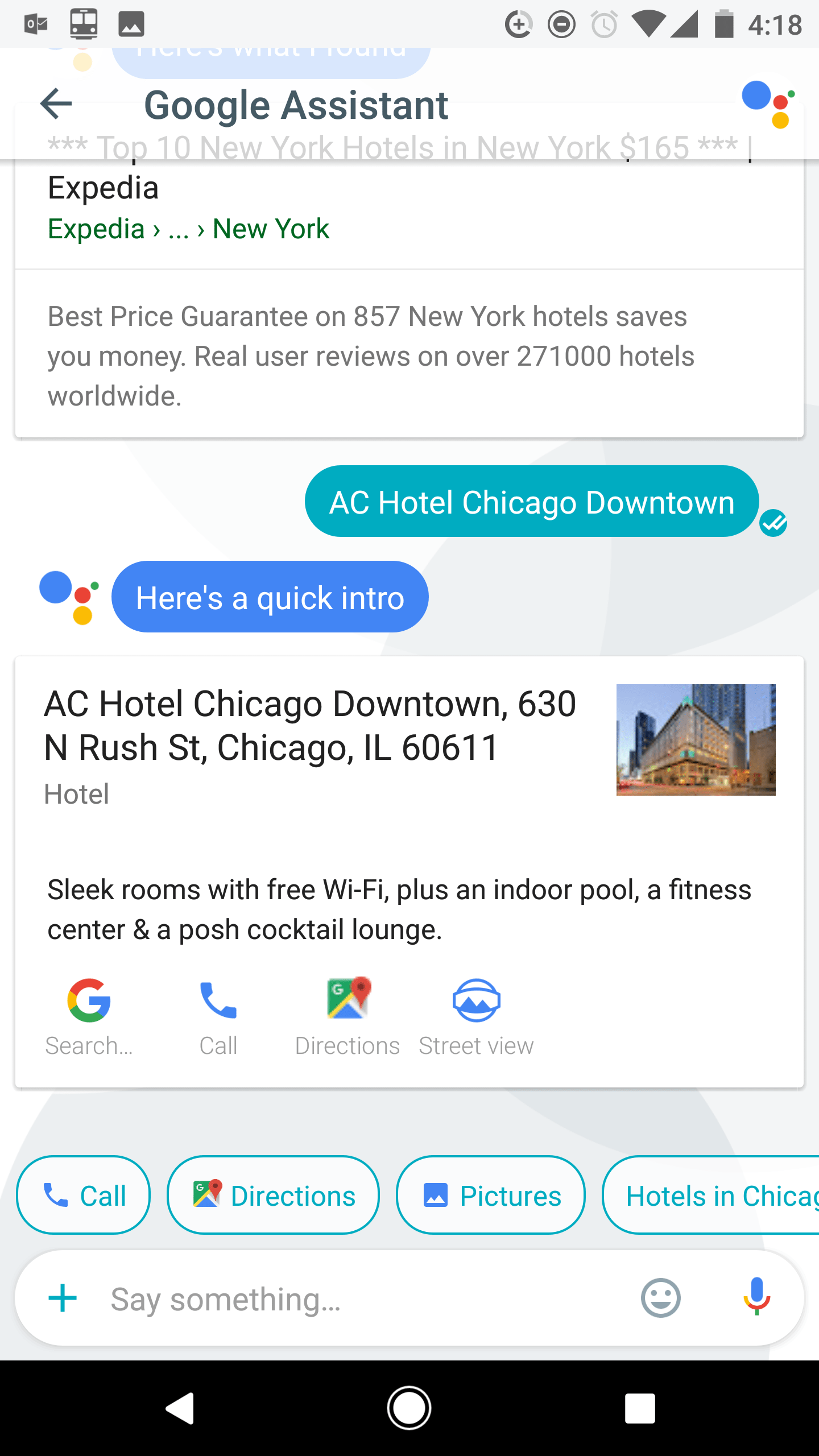A smartphone screenshot in portrait format is captured at 4:18 PM with a battery life of approximately 90-95% and full network reception. The screenshot reveals the Google Assistant app actively displaying information brought up via the user's input. The top of the screen displays typical smartphone interface options, an Outlook notification, and an "Images" icon, indicating these apps are running in the background. 

The main content of the screenshot is centered on a query to Google Assistant about “AC Hotel Chicago Downtown.” Google Assistant has responded with a brief description and details about the hotel, located at 630 North Rush Street, Chicago, Illinois, 60611. The hotel is described as having sleek rooms with free Wi-Fi, an indoor pool, a fitness center, and a posh cocktail lounge. Below the description, there are interactive options such as Search, Call, Directions, and Street View for further exploration of the hotel. Additionally, Expedia's advertisement touts a best price guarantee on New York hotels, emphasizing real user reviews and significant saving offers. 

The detailed and dynamic display of information provides a seamless user experience in exploring potential accommodations through Google Assistant.